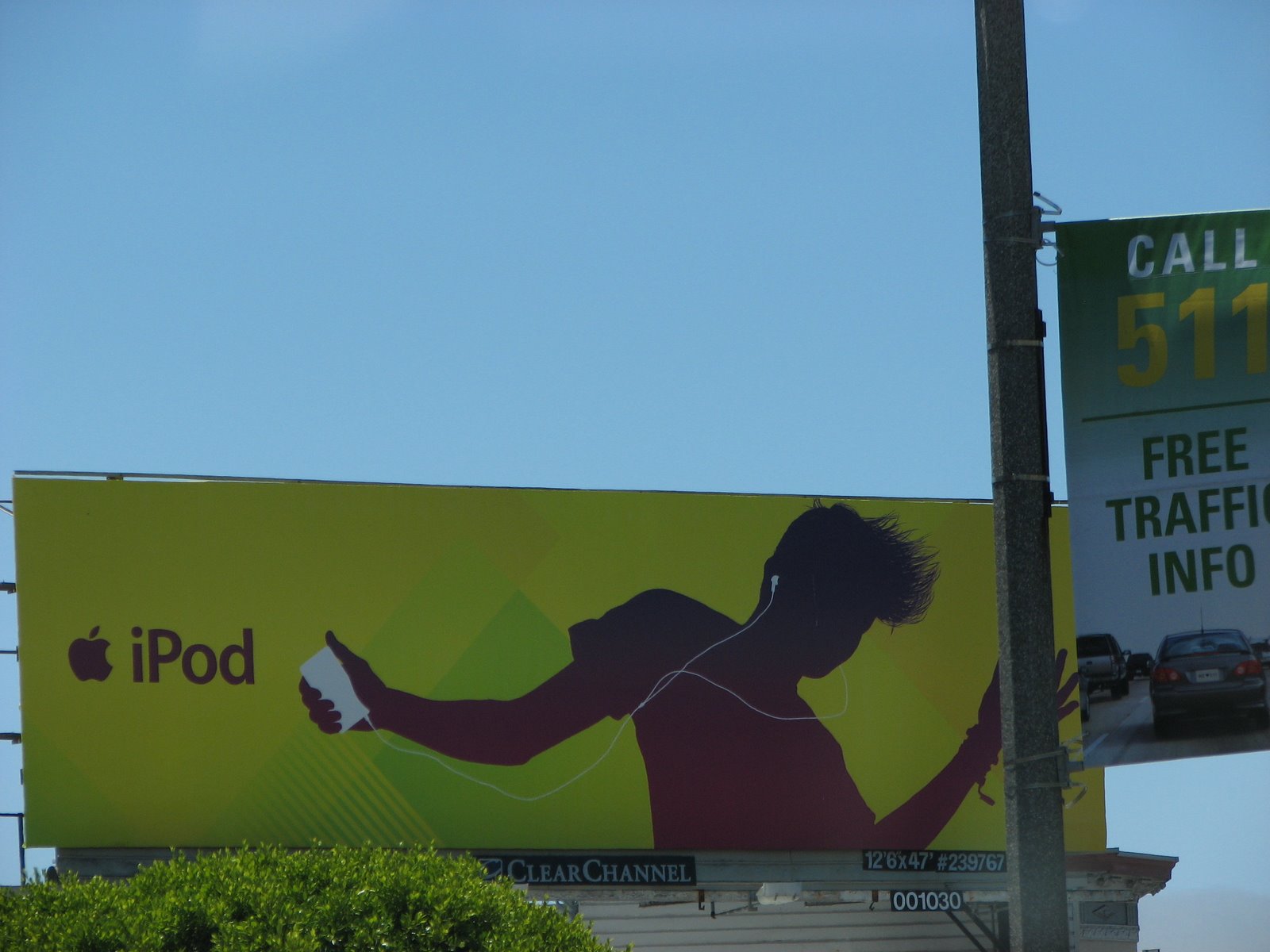This landscape-oriented photograph captures a transitional outdoor scene as the day edges towards dusk, with a gradually deepening blue sky. Dominating the right side of the image is a tall light post, which extends beyond the upper and lower frame boundaries. Attached to the light post is a sign reading "Call 511 Free Traffic Info." Adjacent to the light post is a prominent yellow billboard advertising Apple iPods. The billboard features a silhouetted figure holding an iPod in their left hand, with wired earbuds connecting to their ears, depicted in striking black contrast. Beneath the advertisement is the logo for Clear Channel, along with various measurement information and numbers. In the foreground, a patch of bushes occupies the lower left corner, adding a touch of greenery to the urban setting.